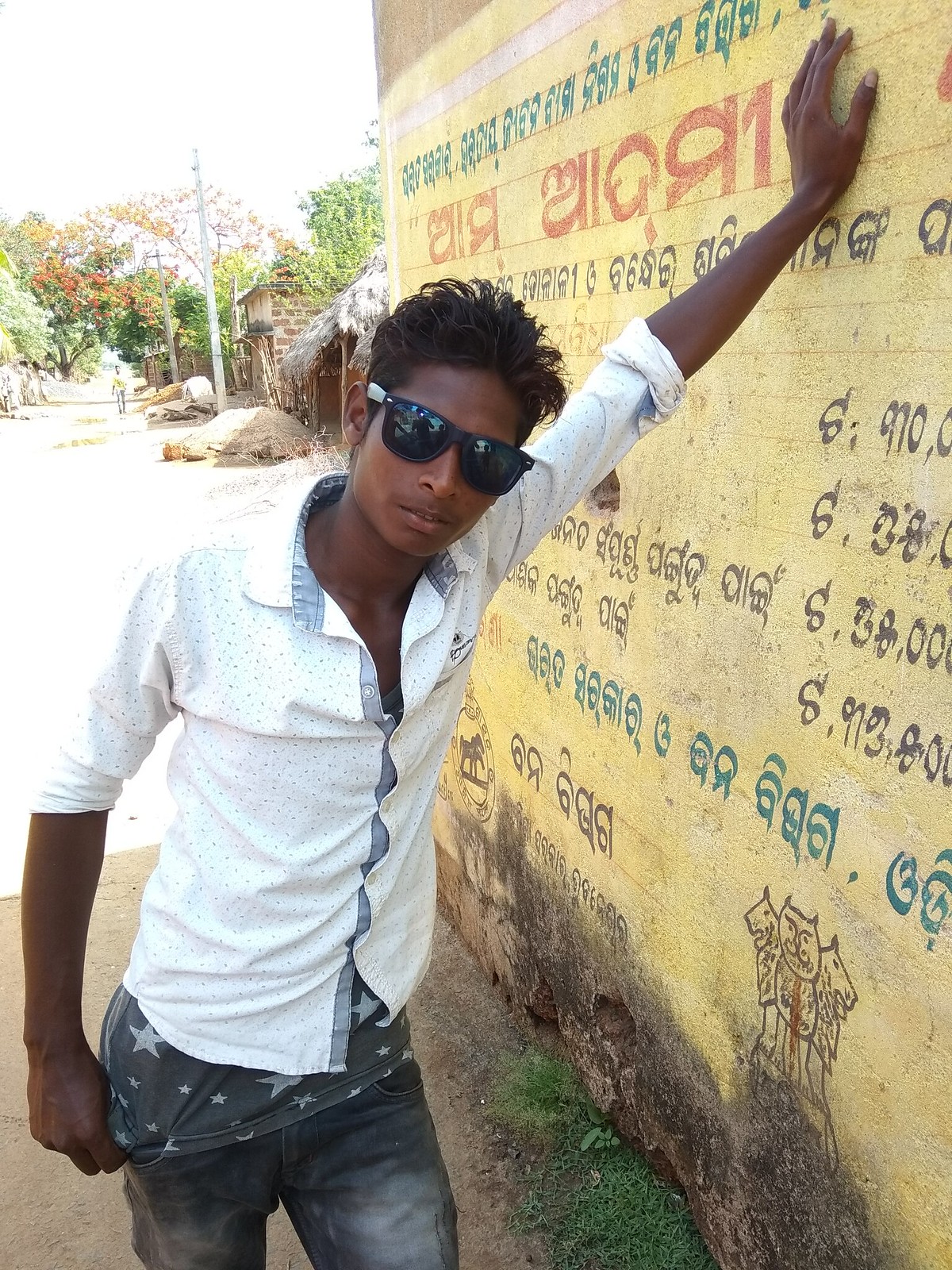This image features a young man in his 20s, striking a pose with his left hand against a wall covered in foreign lettering, including what appears to be oriental characters. The wall is a mix of yellow and red hues with dark brown at the bottom. He sports big black sunglasses and has spiked, medium-length black hair tilted slightly to the right. The man's outfit includes a white jacket with one button near the neck open, revealing an underlayer blue shirt adorned with white stars. He is also wearing stone-washed denim jeans, cut off above the knees in the photograph. In the background, there is a patch of green grass, dirt, a road lined with trees, and a brick building. The overall composition suggests he is leaning casually, exhibiting a fashionable yet laid-back demeanor.